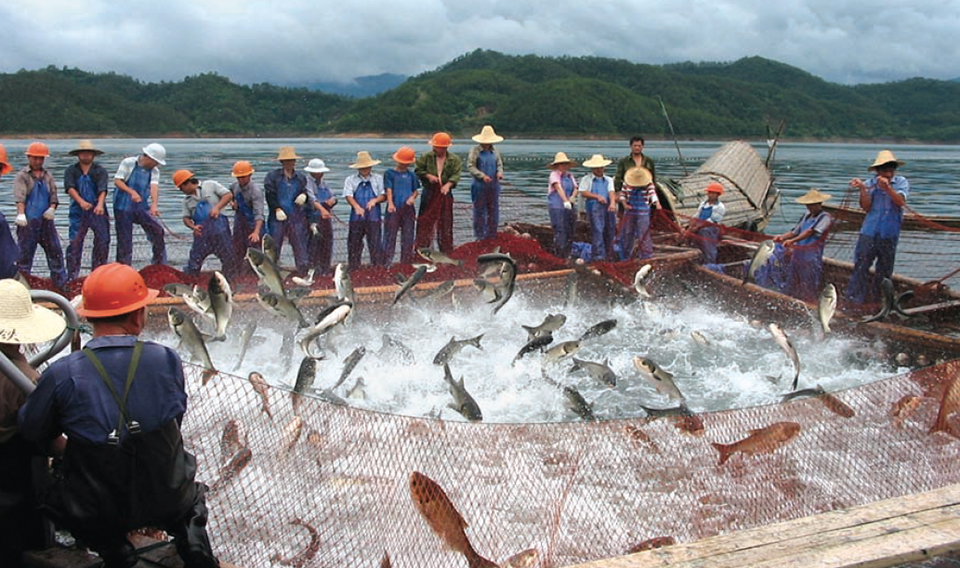The image depicts a busy scene of commercial fishing in a partitioned-off area of water, set against a background of green hills and a cloudy sky. The water, possibly part of a lake or river, is sectioned off with a mesh fence that forms a makeshift enclosure, aided by small boats on one side. The enclosure is brimming with silvery fish leaping out of the water, creating splashes and movement. In the foreground on the bottom right, there's a wooden structure, possibly a dock, and people are positioned around the enclosure. The individuals, some in orange or white hard hats and others in straw hats, are either on boats or standing along the boundary, all seemingly engaged in the fishing activity. The sky above is predominantly gray with scattered clouds, and there's a glimpse of open water and green hills in the background, adding to the natural ambiance of the scene.